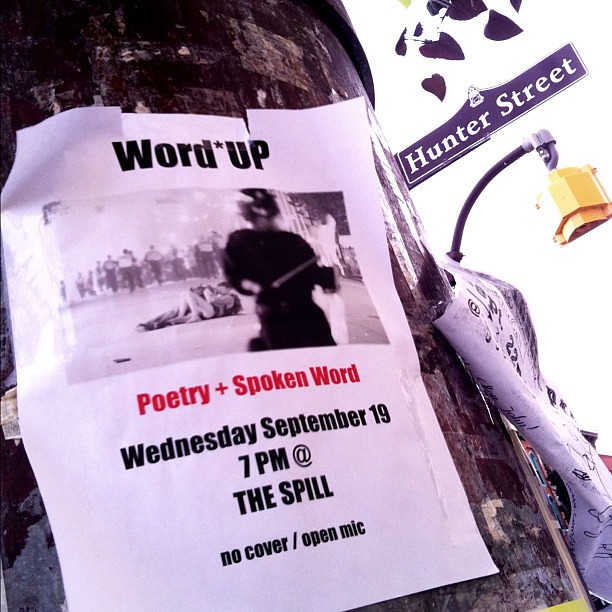A square image captures a cylindrical pole, likely metallic or wooden, that dominates the frame from the bottom right corner, ascending diagonally left. The pole is partially cut off at the left edge and top left side of the image. A white piece of paper, slightly tilted and affixed with clear tape, serves as a makeshift poster on the pole. This poster is somewhat damaged with two rips at the top. Bold black letters at the top of the paper read "WORD UP." Below this, a black-and-white photograph depicts several police officers in the distance, with a couple kissing on the ground in the foreground. Underneath the photograph, red font declares "POETRY PLUS SPOKEN WORD," followed by black text detailing the event: "Wednesday, September 19, 7 p.m. at The Spill, NO COVER / OPEN MIC" with "The Spill" in all caps. The pole could be either a tree trunk or a utility pole, suggested by a nearby sign reading "Hunter Street," a black pipe with a silver top and a yellowish end. The outdoor setting also includes a partial view of buildings and other signs or advertisements, one of which is crumpled and partially blown away.